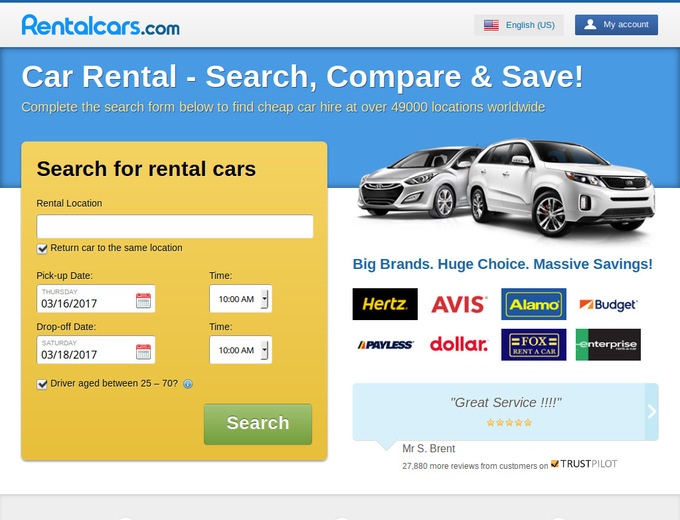The image is a screenshot of the car rental website, Rentalcars.com, displayed on a desktop or laptop screen. The top section features a navigation bar with a predominantly white background and the website's logo, 'Rentalcars.com,' in blue. To the right of the logo are language settings showing 'US English' and an option to access 'My Account.'

Below the navigation bar, a blue banner with white text showcases the website's slogan: "Car rental, search, compare, save!" This is accompanied by a yellow-highlighted instruction urging users to "Complete the search form below and find a cheap car hire at over 49,000 locations worldwide."

The main content area shows a visual of two vehicles: a white 4x4 and a silver sedan. Overlaid text asserts, "Big brands, huge choice, massive savings." The website proudly lists partnering rental companies, including Hertz, Avis, Alamo, Budget, Payless, Dollar, Fox Rent A Car, and Enterprise.

The search form is prominently displayed, featuring fields to specify rental and return locations, pick-up and drop-off dates and times, and the driver's age range (25 to 70 years). A green 'Search' button with white text invites users to begin their car rental search.

A testimonial from a Trustpilot user, Mr. S. Brent, is featured at the bottom of the search form. It reads, "Great service!!!" and is accompanied by a five-star rating.